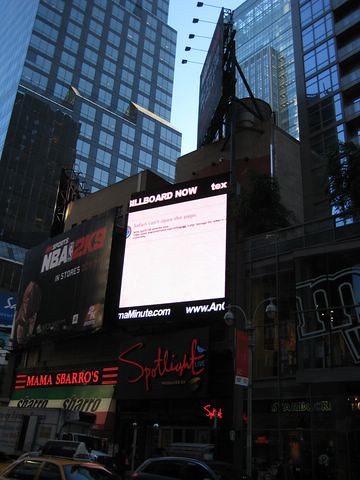The image depicts a bustling urban scene, focusing on a side of a building in a city environment. At the bottom of the frame, the tops of two vehicles are visible, positioned side-by-side. On the left, a brown vehicle is seen, while on the right, a gray vehicle appears.

Above the vehicles, the facade of a building is adorned with several signs. On the lower left side, there is a sign with the text "Mama Barrow's" in red. To its right, there's a black sign with cursive red text reading "Spotlight". Further up the building, a square-shaped billboard comes into view, featuring black sections with white text at the top and bottom, and a plain white screen in the center. Adjacent to this, on the left, is another black sign displaying "NBA 2K9", with "NBA" in white and "2K9" in red letters. At the very top, the building is capped with a brown section.

Flanking this central building are two tall structures, each with distinct features. On the left, a multi-story building boasts a light blue and gray color scheme. Meanwhile, the building on the right is characterized by its extensive glass windows.